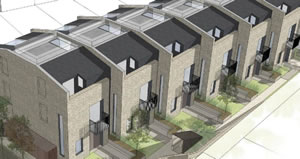This image appears to be a detailed digital rendering of a row of six small, light brown brick townhomes, possibly mistaken initially for concrete structures. The view is from above and at an angle, showing that these homes, which might also serve as commercial storefronts, are staggered in design. This offset layout creates a cascading effect from left to right. Each townhome has a gray and black angled roof, some of which suggest the presence of skylights or solar panels. Every unit features its own yard adorned with greenery, a small walkway, a front door beside a column, and a balcony. The street view includes trees interspersed between the buildings and additional walkway paths in front and back of the units. The scene is overcast, adding a subdued tone to the overall ambiance. Additionally, each apartment has external lights and windows strategically placed between the door and column, enhancing both function and aesthetic appeal.